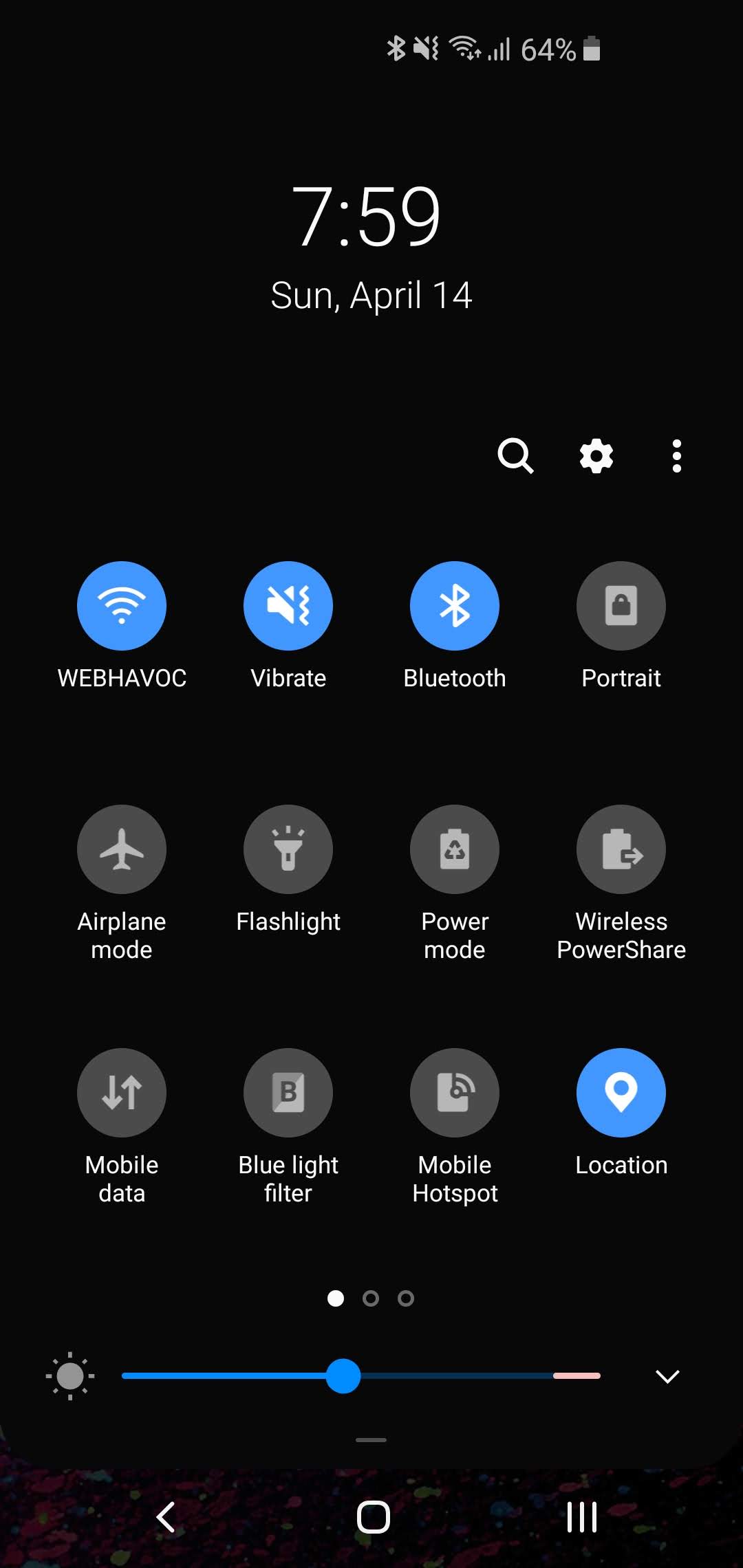The image displays a cell phone screen featuring various status icons and settings options. 

### Detailed Caption:

The cell phone screen showcases an array of icons and settings predominantly in black, white, gray, and blue hues. At the top middle-right of the screen lie the status indicators: Bluetooth, no sound, vibrate mode, Wi-Fi signal bars, cellular signal bars, and a battery icon showing 64% charge. Centered just below these icons is the current time, displayed as "7:59," along with the date "Sunday, April 14th."

To the right of the time and date are three icons: a search icon, a settings gear icon, and a vertical ellipsis (three dots stacked). Below, a grid layout presents four rows of apps, each containing four icons. The upper left app icon is labeled "Web Havoc." Next to it along the first row and successive rows are icons for vibrate, Bluetooth, portrait mode, airplane mode, flashlight, power mode, wireless power share, mobile data, blue light filter, hotspot, mobile hotspot, and location services.

Beneath this grid are three dots, indicating multiple pages of settings options, with the first dot highlighted, suggesting the current view is the first page. Further down is a horizontal slider bar featuring a bright sun icon on the left and a downward arrow on the right, likely representing screen brightness control. At the very bottom of the screen, there are navigation icons for the phone: a left-pointing arrow, a circle, and three horizontal lines, typically used for back navigation, home, and recent apps, respectively.